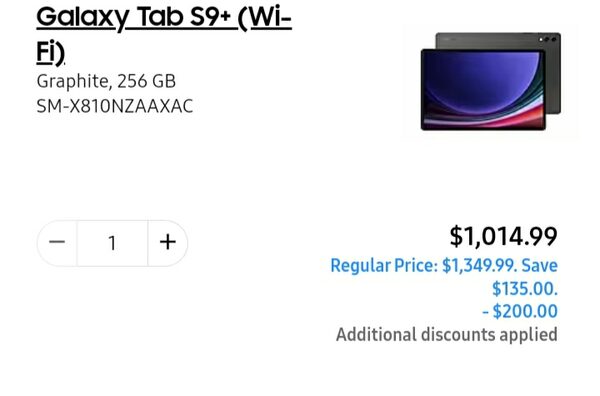This image is a detailed screenshot from an undisclosed webpage showcasing the Galaxy Tab S9+ in graphite with 256 gigabytes of storage and the model number SM-X810NZAAXAC. The background is plain white. At the top left corner, the product name and specifications are clearly displayed. Below, there is a quantity selector with a minus sign on the left, a '1' in the center, and a plus sign on the right. In the top right of the image, there is a photograph of the Galaxy Tab S9+, showing both the graphite gray back and the front screen featuring an abstract shapes wallpaper. The price is prominently displayed as $1,014.99, marked down from the regular price of $1,349.99, indicating a savings of $135 along with an additional $200 discount. The image is purely product-focused and contains no other elements such as people, animals, birds, fish, plants, flowers, trees, buildings, bridges, or automobiles.